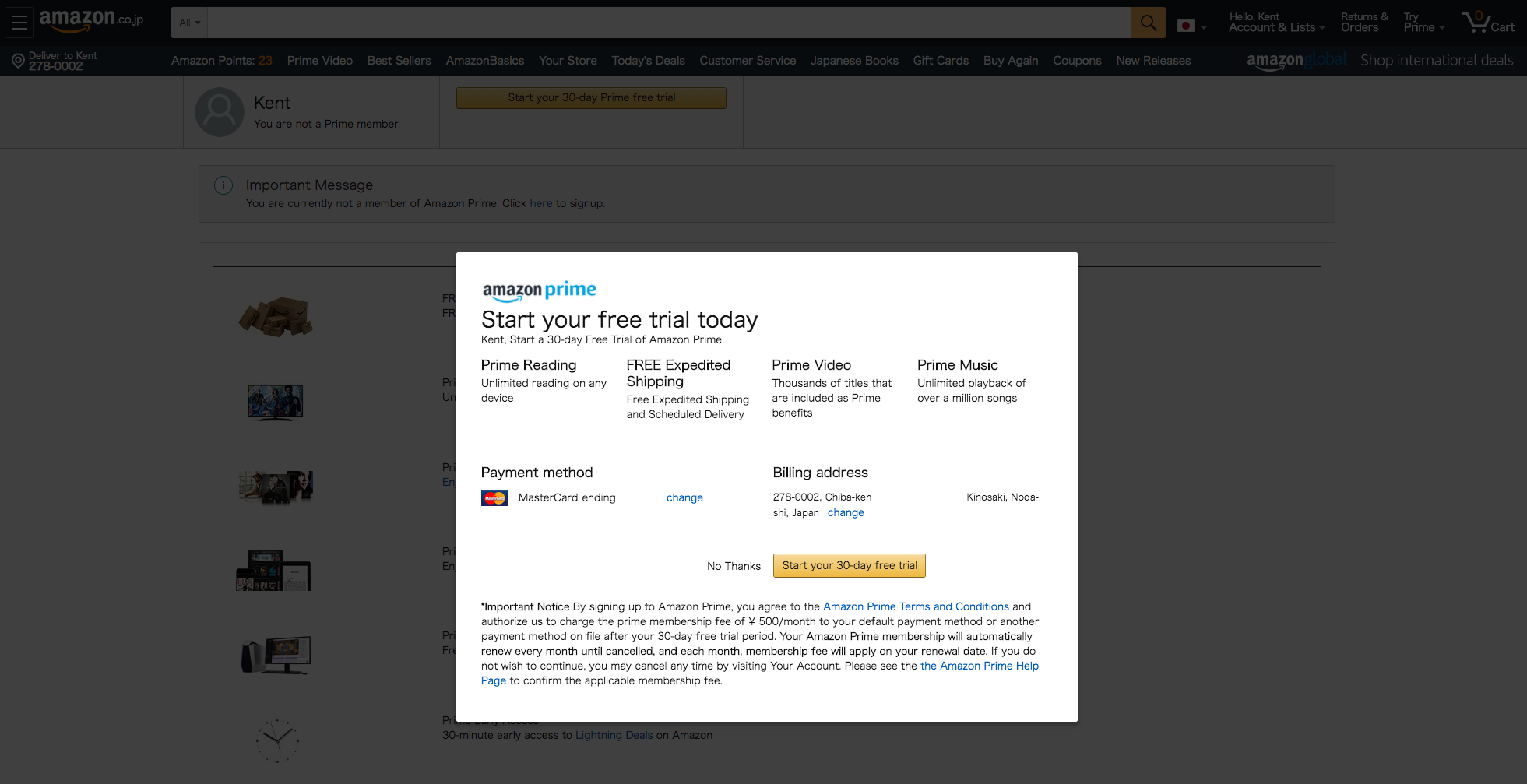In this rectangular image, we are viewing a screenshot of an Amazon webpage. The background is a dark gray, and prominently displayed on top is a large white rectangle. Within this rectangle is text promoting Amazon Prime and its benefits. The headline reads, "Amazon Prime, start your free trial today." Below that, it invites Kent to begin a 30-day free trial of Amazon Prime, detailing various benefits such as "Prime Reading – unlimited reading on any device," "Free expedited shipping and scheduled delivery," "Prime Video – thousands of titles included as Prime benefits," and "Prime Music – unlimited playback of over a million songs."

On the left side of the image, there is a section for payment and billing information, which includes a MasterCard ending and the billing address: "278-0002 Chibaken, Chi, Japan, Kenosuke Noda." At the bottom of the white rectangle are two options for the user to choose from: "No thanks" and "Start your 30-day free trial."